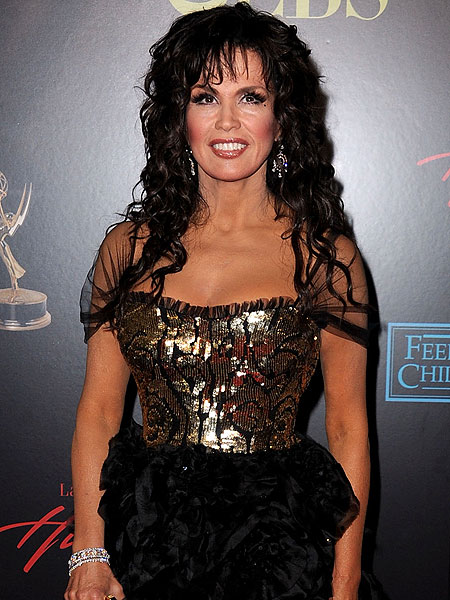The image depicts an older woman, possibly in her 50s or 60s, posing for a photo at what appears to be a red carpet event or awards ceremony, possibly the Golden Globes, indicated by the backdrop featuring partially cut-off signage that includes a CBS logo and an award image. She has long, wavy black hair with bangs and is wearing a sparkly golden top with detailed mesh see-through shoulders. Her outfit includes a ruffled black skirt, and she accessorizes with a bracelet and shiny earrings. The woman, who looks rather tan and is wearing heavy makeup including blush, eye makeup, and lipstick, stands facing the camera with her arms at her sides, smiling or attempting to smile directly into the lens.